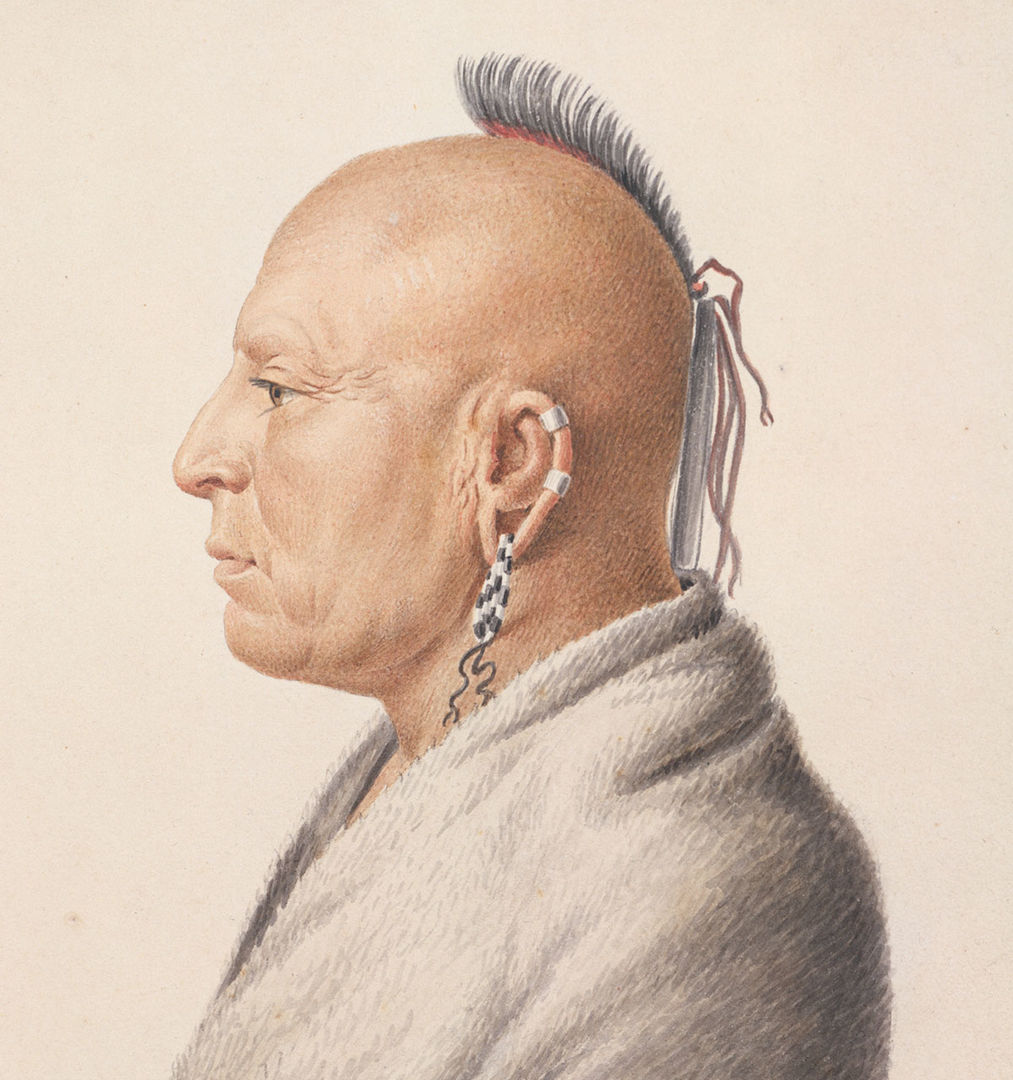This detailed painting depicts a Native American man in profile, facing left. His head is mostly bald, except for a striking black mohawk that originates farther back on his scalp and extends down, tied with brown leather strings into a long strand at the back. Adorning his left ear are two silver hoop earrings and a beaded dangle on his earlobe. He wears a white terrycloth coat, reminiscent of a robe or a fine fuzzy blanket, draped around his shoulders. The background is rendered in a simple, off-white color, drawing attention to the subject's distinctive features, such as his prominent nose and heavy jowls.